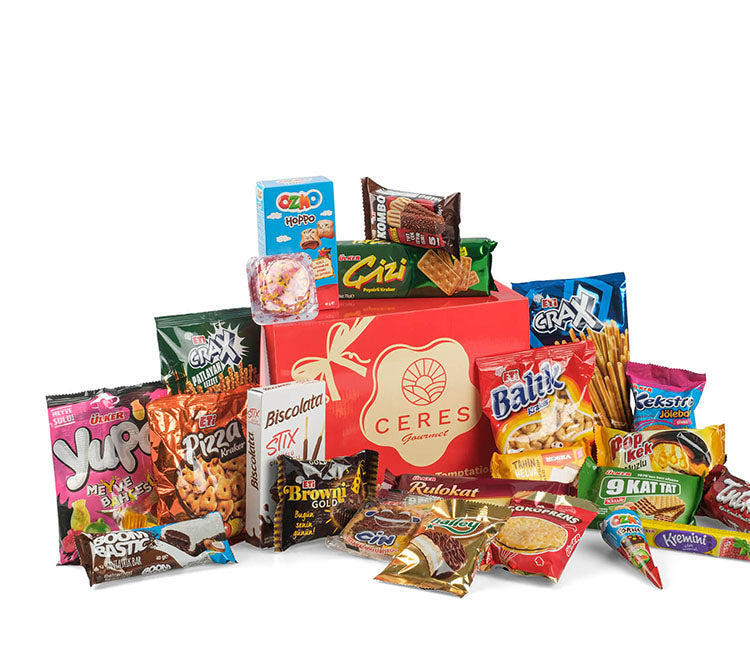The image depicts an assortment of approximately 15 to 20 vibrant and uniquely packaged snack foods, likely from a snack subscription or delivery service. Dominating the center of the photo is a large red box labeled "Ceres Gourmet," set against a clean, white background. Surrounding the box are various types of snacks, including cookies, pretzels, crackers, and chocolates, as well as some savory items like flavored chips and pizza crackers. Most packaging features intriguing designs and a rainbow palette of bright colors—pinks, reds, purples, greens, and blues. The snacks' labels are mainly in a language other than English, suggesting international origins. Reflective packaging gleams under probable studio lighting, enhancing the appeal. Specific items identified include Biscolada Sticks, a bag of pizza crackers, mini pies, and treats akin to pretzels and brownies. This image, likely intended for advertising, showcases a diverse and colorful range of snacks from around the world.